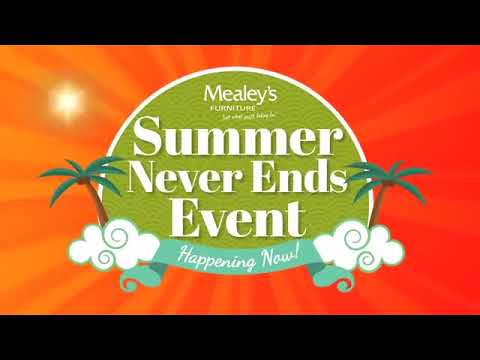This image is an advertisement for "Miele's Furniture," promoting their "Summer Never Ends Event." The design features black bars at the very top and bottom, with a vibrant background that transitions from a light to medium orange gradient accented by sun rays emanating from the center. A subtle sun flare is positioned on the upper left. The central part of the advertisement displays a textured medium green semicircle with a white border. Inside the semicircle, white text prominently states "Miele's Furniture," followed by the event name in cursive, "Summer Never Ends Event." This text is bordered by a light blue ribbon at the bottom displaying "Happening Now!" in white letters. Flanking the blue ribbon are illustrations of clouds with palm trees emerging from either side. The color scheme enhances the summery feel of the advertisement, effectively highlighting the ongoing furniture event.